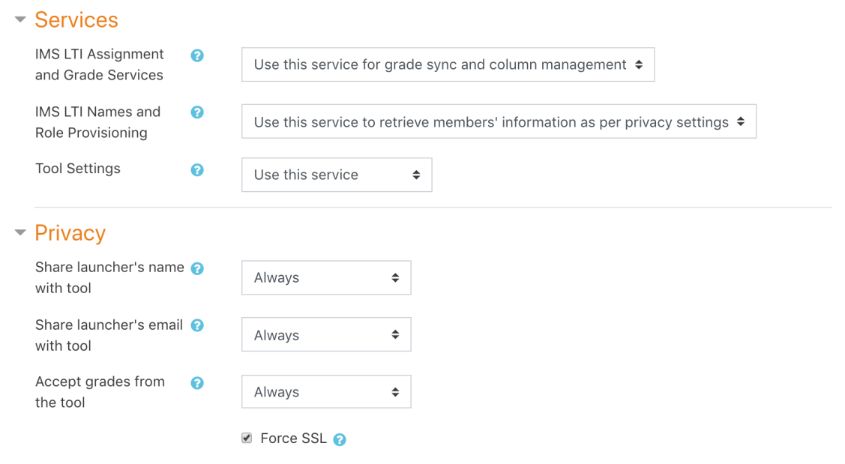This image depicts a screenshot of a web page, primarily detailing various service and privacy settings. At the top, a drop-down menu labeled "Services" is visible, which includes options such as IMS, LTI Assignment and Grade Services. Adjacent to this, a box advises, "Use this service for grade sync and column management."

Below these options, there is a listing for "IMS, LTI Names and Role Provisioning," accompanied by an instruction box stating, "Use this service to retrieve members' information as per privacy settings." Further down, the "Tool Settings" option is displayed, alongside a succinct message urging users to "Use this service."

Moving towards the bottom section, the "Privacy" settings are prominently featured. These include:
- "Share launcher's name with tool," which has an associated box set to "Always."
- "Share launcher's email with tool," also accompanied by a box set to "Always."
- "Accept grades from the tool," similarly configured with a box set to "Always."

Finally, at the very bottom, there is an option labeled "Force SSL," which is checkmarked, indicating it is enabled.